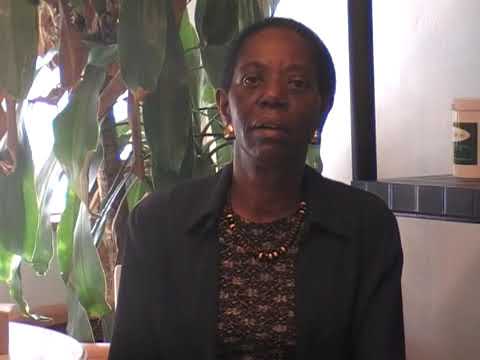A black woman is centered in the image, staring straight forward with a look of despair on her face. Her brown eyes are open, and her hair is short, pulled back behind her head. She is wearing small gold earrings and a black collared over-shirt with a dark-colored floral-patterned undershirt. Around her neck is a brown and gold beaded necklace. Her mouth is slightly open, revealing the bottom of her top teeth. The background includes some green and brown leaves hanging down from the ceiling on the left, while on the right side above her shoulder, there is a tiled surface with a light pink bottle featuring a green label. The image quality is somewhat pixelated, suggesting it might be a screen capture from a stream or video call. The room appears to have white walls, and beyond the plants, there might be a white and brown container visible.